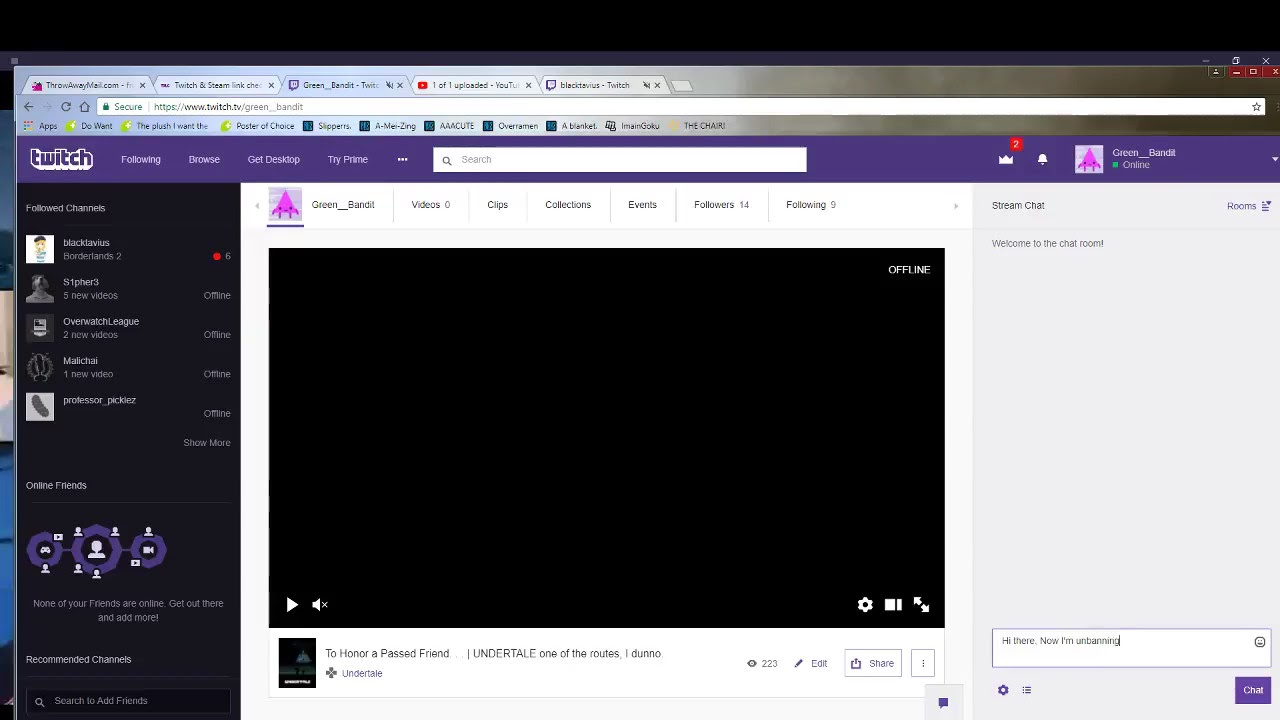Screenshot of a Twitch Website

The screenshot captures a webpage of the Twitch website. The main body of the site is painted in a light gray background, while the top navigation bar features a distinct purple hue. On the left side, a black sidebar adds depth to the layout.

At the top of the screenshot, one can observe five open browser tabs, though the labels are unreadable due to the small size of the image. In the top left corner of the purple navigation bar, the "Twitch" logo stands prominently, with white text and a purple background. Adjacent to the logo are four menu options in white against the purple bar followed by a centrally placed search bar. Farther to the right, the account login details and user settings are located.

The left sidebar, painted in black, displays avatars of five different people. Below these avatars are three purple circles, each featuring a white silhouette of a head and shoulders, indicating user icons. Due to the image's resolution, additional details about these icons are unclear.

Centered on the main page, there is a black screen placeholder for a video, indicating that the content has not yet loaded. Positioned at the bottom of this screen are the playback control icons: a play button in the bottom left corner, a speaker icon for volume control, a settings cog, and an expand icon in the bottom right. The remaining details in the screenshot are too small to decipher.